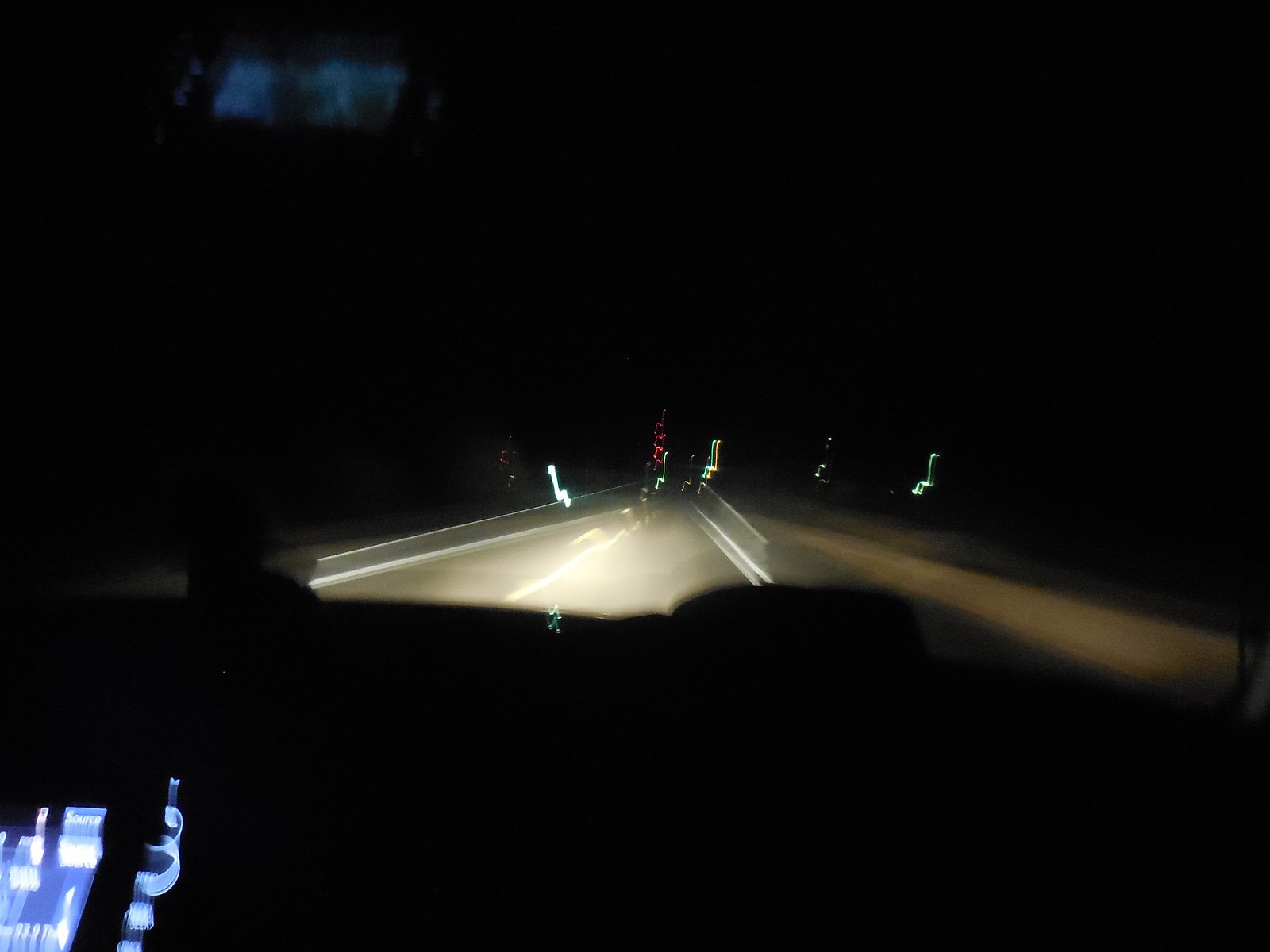The image captures a nighttime view from the interior of a vehicle, gazing out at the road illuminated by the car's headlights. Inside the vehicle, in the corner of the image, there is a segment with blue writing, likely from the dashboard or a digital display, though the text is blurred and hard to discern. The scene beyond the windshield reveals a road bordered by two areas bathed in light that create shapes resembling chairs, positioned on either side of the road. Further ahead, there is a small, indistinct spot that has a hint of red coloration, but like much of the view, it remains out of focus.